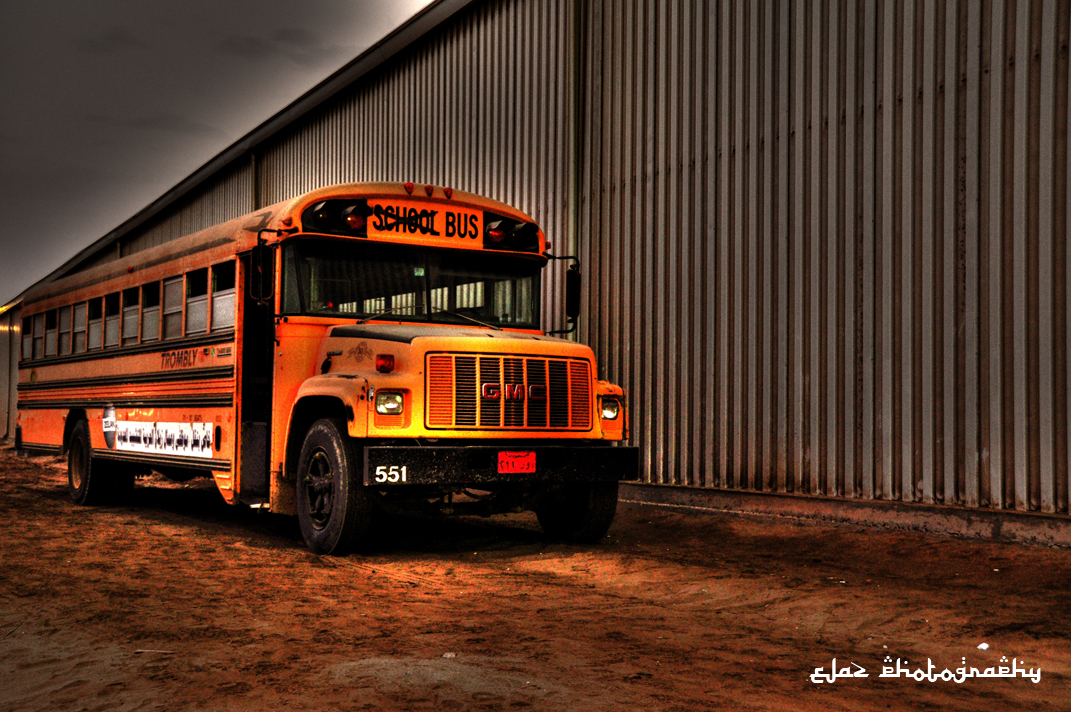In a surreal and dimly lit setting, a glowing yellow-orange school bus stands prominently within a large, metallic-walled garage or warehouse. The bus, a classic GMC model, is positioned left of center and viewed from the front and right side in a three-quarter perspective. The word "SCHOOL" on the placard above the windshield has been conspicuously crossed out with a black X, leaving only the word "BUS" legible. The bus bears the number "551" in white on its red license plate at the bumper's left corner.

Emblazoned along the side of the bus is the word "Trombly," alongside a long white decal just above the bottom of the chassis, extending about a third of the bus's length. The bus doors are open, suggesting an abandoned or inactive state. The floor beneath consists of a black and brown marbled pattern, and the surroundings are a mix of uncovered dirt and the reflective, corrugated iron walls of the warehouse. Adding an enigmatic touch, there is non-English script, possibly Arabic, written in the lower right corner of the image.